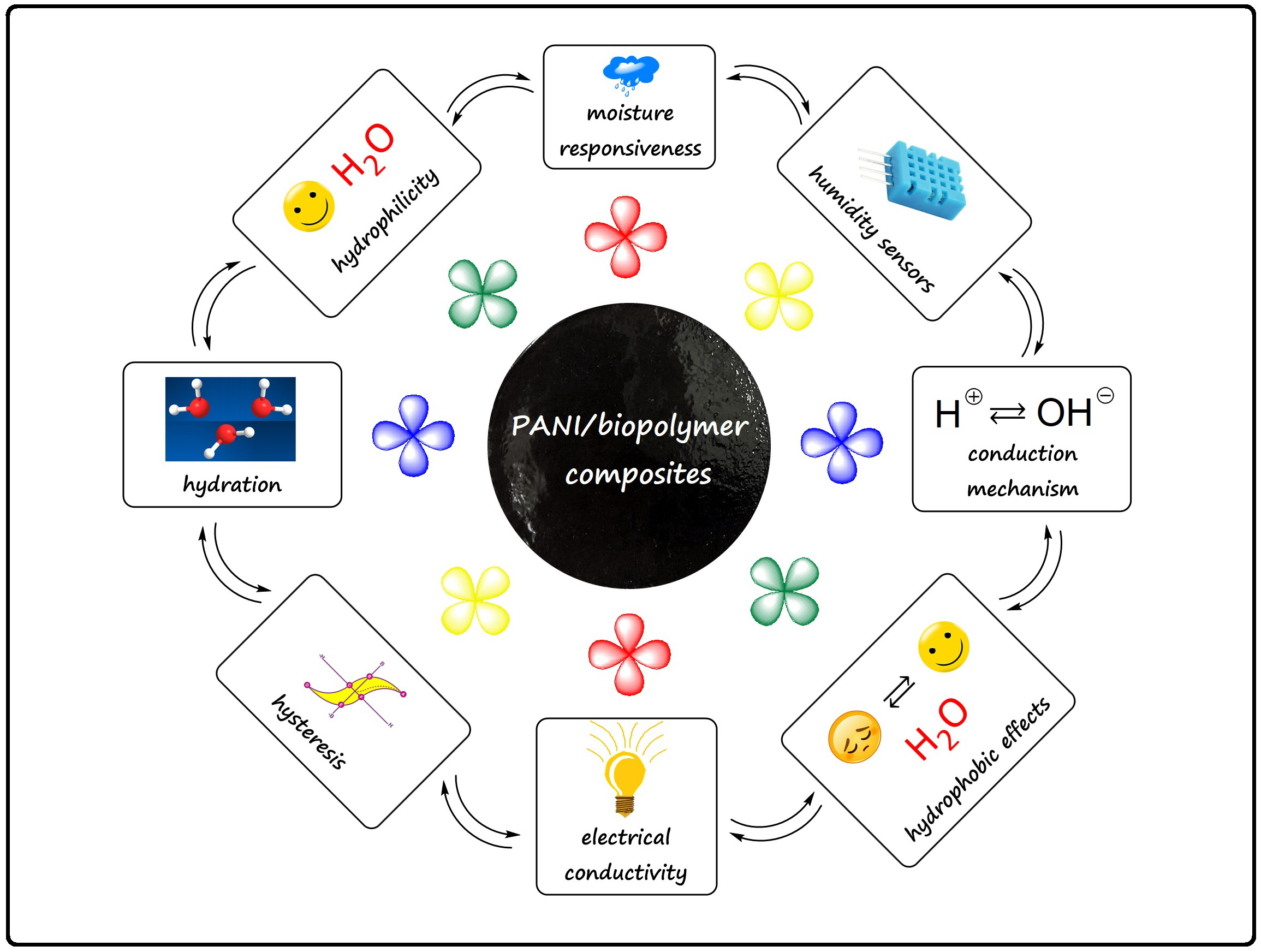The image is a detailed schematic depicting a scientific process involving moisture and conductivity properties of materials, particularly focusing on PANI (Polyaniline) bi-polymer composites. The central feature is a black sphere with white text that reads "PANI/Bi-Polymer Composites," surrounded by colorful flower-like shapes in red, yellow, blue, and green. Arranged in a circular layout around this central sphere are multiple black-outlined rectangles and squares, each containing text and images related to humidity sensors, moisture responsiveness, hydrophilicity (with a smiley face), hydration, and electrical conductivity (illustrated with a light bulb). These rectangles are interconnected by arrows indicating a bi-directional, equal exchange of information or processes, illustrating the complex interplay between these factors. The entire diagram is set against a white background with a black border, enhancing the clarity and focus on the presented information.